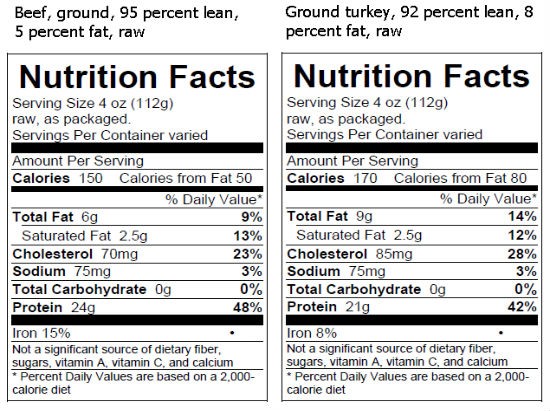This image showcases a comparison of the nutrition facts for two different products, ground beef and ground turkey. The information is presented within a black outline box, featuring black text on a white background. The nutrition labels are placed side-by-side for easy comparison, with ground beef on the left and ground turkey on the right. 

Above the nutrition facts for the ground beef, the text reads "Beef, Ground, 95% Lean, 5% Fat, Raw." Similarly, the text above the ground turkey label states "Ground Turkey, 92% Lean, 8% Fat, Raw." 

Both labels follow the same layout, providing detailed nutritional information, including metrics such as calories, fat content, cholesterol levels, and other relevant data. This detailed side-by-side comparison allows for a clear understanding of the nutritional differences between the two types of ground meat.